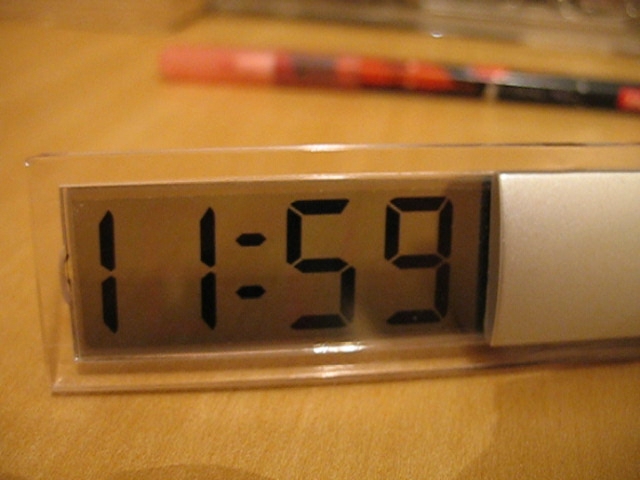This photograph features a clear acrylic digital clock prominently displaying the time as 11:59 in bold black digits against a grey background. The clock's minimalist design is complemented by a white panel situated on top of it. This entire setup rests on a wooden table or desk, adding a natural element to the scene. In the background, slightly out of focus, a red cylindrical object can be seen. This object, possibly a pen or pencil, introduces a contrasting pop of color with its red body and black detail, further enhancing the composition of the image.